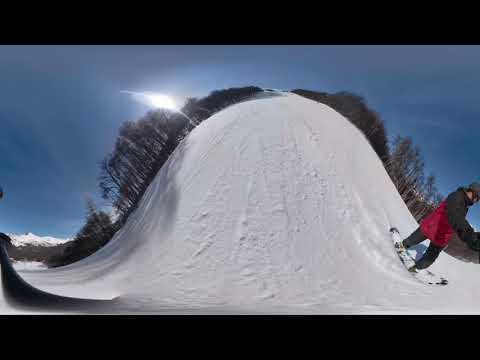The image captures a serene snow-covered landscape dominated by a gently sloping hill, which appears larger and more rounded due to a fisheye lens effect, resembling the top of a mushroom. The hill is blanketed in thick, pure white snow, with a snowboarder descending its slope. The snowboarder is outfitted in a gray helmet, red and black jacket, black snow pants, and is riding a white snowboard. The vibrant blue sky overhead is cloudless, enhancing the crispness of the scene. Flanking the hill are rows of bare trees, devoid of leaves, adding a stark contrast to the snowy expanse. In the lower left background, there is a higher mountain topped with craggy rocks and snow, creating a dramatic backdrop. The sun is visible in the top left horizon, further illuminating this winter wonderland.